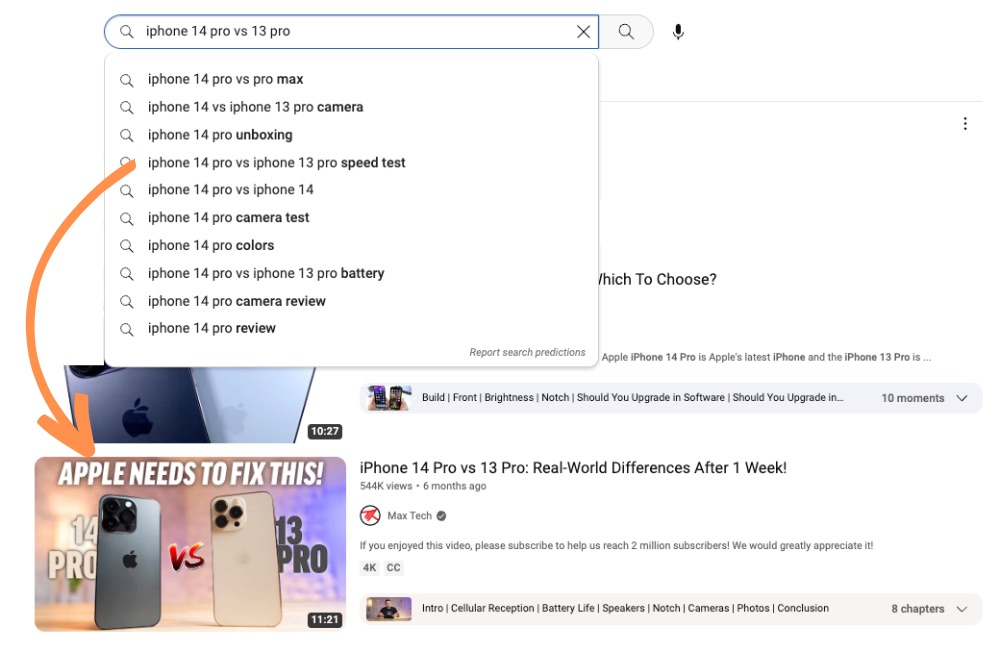The image depicts a YouTube search query for "iPhone 15 Pro versus 13 Pro." Below the search box, YouTube suggests several related searches, including "iPhone 14 Pro versus Pro Max," "iPhone 14 versus iPhone 13 Pro camera," "iPhone 14 unboxing," "iPhone 14 Pro versus iPhone 14 Pro 13 Pro speed test," along with various other suggestions pertaining to iPhone comparisons and reviews.

On the left side of the screen, there's an orange error indicator pointing to the second video thumbnail, which is located at the bottom left. The thumbnail features the text "Apple needs to fix this" and includes images of both the iPhone 14 Pro and the iPhone 13 Pro. This video, titled "iPhone 14 Pro versus iPhone 13 Pro: Real World Differences After One Week," has garnered 544k views and was uploaded six months ago by Max Tech.

In the background, the first video displayed is titled "Which to Choose: Build, Front, Brightness, Notch, Should You Upgrade the Software?" This video has a duration of 10 minutes and 27 seconds and includes 10 comments. The details of the videos and suggestions aim to inform viewers about the differences and improvements between various iPhone models, particularly focusing on the iPhone 14 and iPhone 13 Pro series.